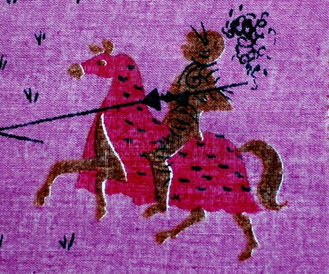The small, square image portrays a knight riding a dark brown horse, adorned with a red blanket that covers its head, body, and has openings for the tail and legs. The background features a dark purple hue interspersed with a few smaller black areas. The knight, donned in armor, sits atop the horse without a visible saddle, gripping a jousting lance. The knight's skin is brown with black stripes, matching the horse's coloration. The blanket features black dashes, lending the image an intricate pattern. Black curls emerge from behind the knight's head, and the scene includes black grass blades on the left side. Additional details suggest a whimsical, storybook-like quality, evoking an image drawn for children's media.